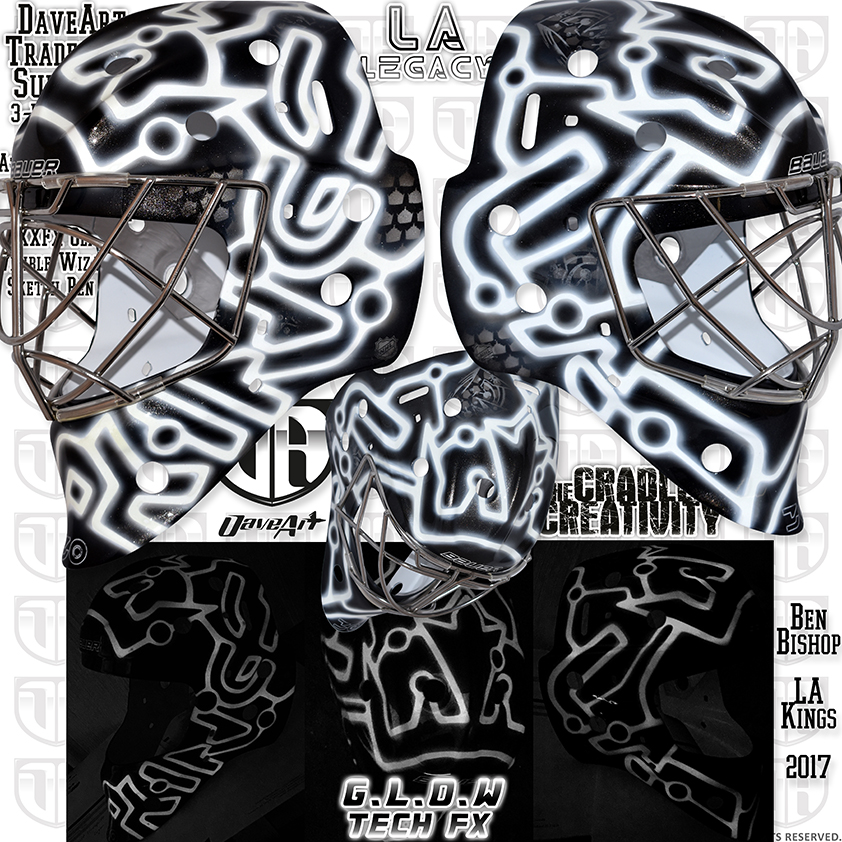The image is a detailed black-and-white poster, primarily featuring two black helmets with intricate white designs positioned at the top and facing away from each other. These helmets resemble those of hockey goalies, complete with metal face guards and neck protection. Between the helmets, "L.A. Legacy" is prominently displayed. Below these helmets, a third helmet faces downward, further adding to the composition. 

In the bottom third of the poster, a black rectangle houses various graphic elements and text. Centered within this section is the acronym "G.L.O.W." in bold black letters with a white border, and beneath it is "TechFX." On the right-hand side within this lower portion, there is a smaller area with additional text in black that reads, "Ben Bishop, L.A. Kings 2017." Partial and obscured text on the left side reads "Dave Art Trade," indicating the artist's credit. The overall aesthetic evokes a blend of street graffiti and artistic design, suggesting a tribute to the sports team or event.